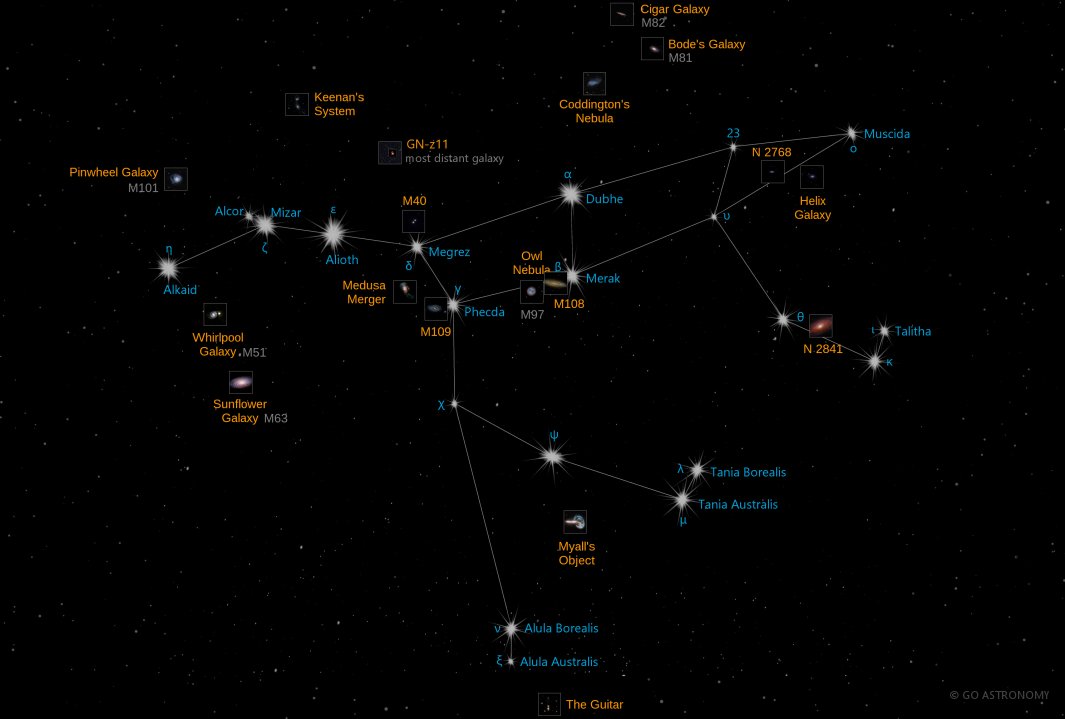This photograph showcases a detailed, annotated diagram of a constellation against a pitch-black night sky, suitable for a magazine or textbook. The constellation, which somewhat resembles a horse, is meticulously mapped out with thin white lines connecting its primary stars. These stars are prominently labeled in blue text, including names like Alkaid, Alcor, Mizar, Alioth, Magrez, Phecda, Merak, Dubhe, Tania Borealis, Tania Australis, Talitha, 23, and Muscida.

Surrounding the constellation are various astronomical objects labeled in orange text, highlighting significant celestial features and systems beyond the immediate constellation. These include the Pinwheel Galaxy, Whirlpool Galaxy, Cigar Galaxy, Coddington's Nebula, Bode's Galaxy, Helix Galaxy, Kenan System, GN-z11, N2841, and M108. Each of these is enclosed in a box, distinguishing galaxies, nebulas, and other stellar phenomena.

The entire image is an intricate blend of photographic realism and scientific illustration, creating a comprehensive guide to this section of the night sky. The detail is from GO Astronomy, ensuring accuracy and educational value.